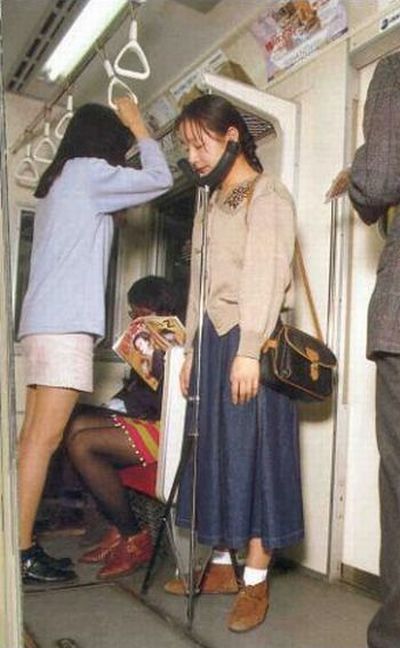In the image, three people are inside a subway car. The central figure is a woman with dark brown hair, pulled back with bangs, standing against the wall. She wears a beige long-sleeve shirt, a blue denim skirt that reaches her shins, white socks, and brown shoes. She has a black and brown purse slung over her shoulder and her chin rests on a gadget that extends to the floor, appearing like a chin rest. To her left, a person with dark skin sits reading a magazine, dressed in red shoes, a red and yellow skirt, and a dark top, and possibly wearing glasses. Nearby, another woman with long dark hair holds onto one of the five white handles hanging from the ceiling. She wears a light blue long-sleeve top, shorts, and black shoes. Additionally, on the far right side, part of a man in a dark gray suit is visible. The overall setting is clearly the interior of a subway car, indicated by the presence of ceiling handles and the typical seating arrangement.